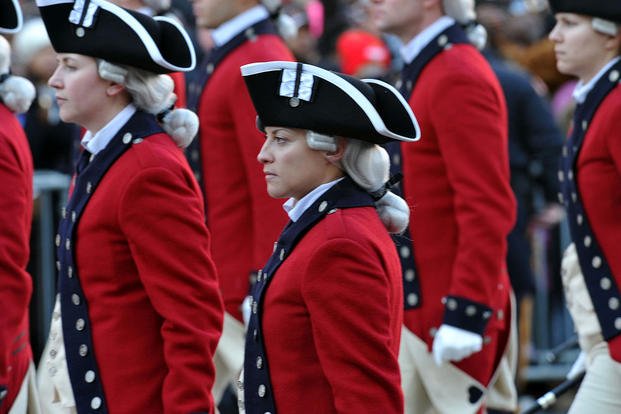This photograph features a group of soldiers, likely British, dressed in historical military uniforms reminiscent of the 1700s. Their attire includes bright red woolen jackets with large collars and blue fabric strips adorned with metallic buttons running down the front, as well as similar detailing on the cuffs. Each soldier wears white gloves and white pants. They also sport traditional black tricorne hats with white trim, and long white powdered wigs that are tied back, forming a bun. The group comprises both males and females, all positioned in a manner suggesting they might be in formation. Their expressions are serious, adding to the historical authenticity and solemnity of the scene.